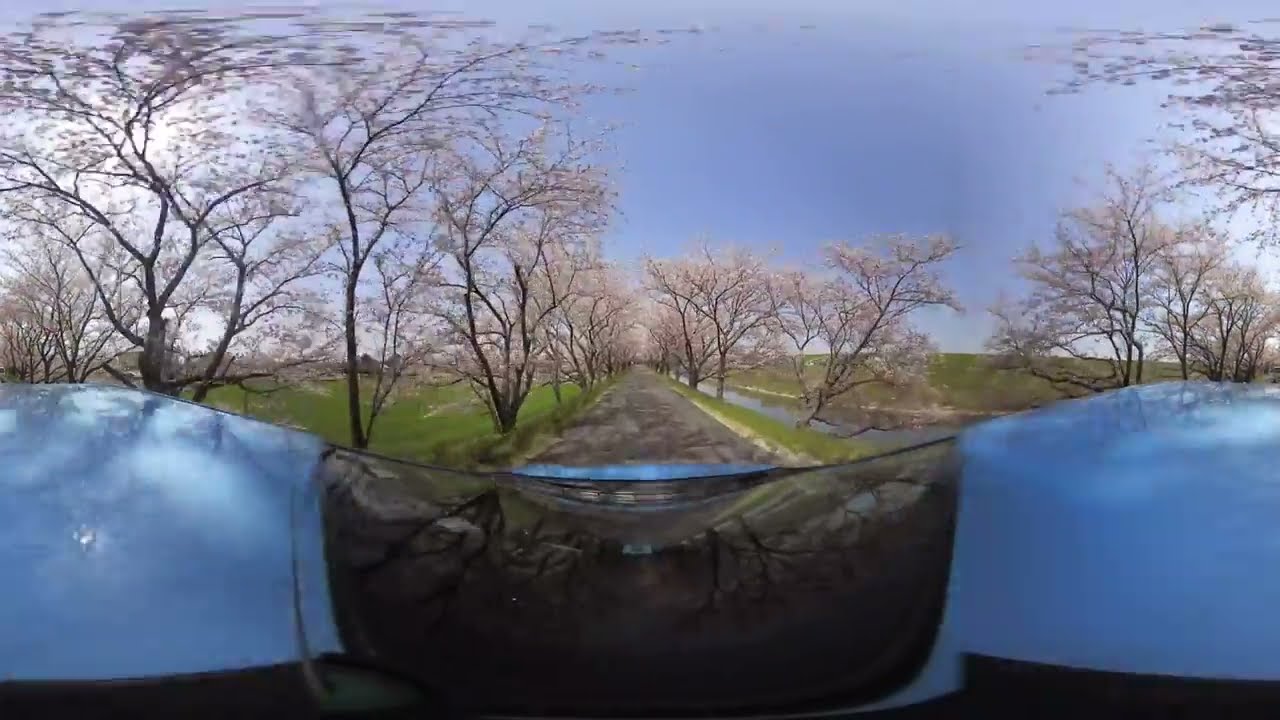The image captures a horizontally aligned, rectangular panoramic view of a picturesque country road. The top half is dominated by a moody sky, adorned with a mix of dark gray and bright white clouds, suggestive of an impending storm. The road itself, positioned centrally, is flanked by tall, flowering trees with light purple blossoms, contributing to a serene yet vibrant scene. The blooming trees, some with bare branches, line both sides of the road, creating a tunnel-like effect. To the right of the road, a narrow strip of water runs parallel, bordered by grassy fields that extend into gently rolling hills. On the left, a larger grassy expanse stretches out, containing a few distant houses. The foreground reveals the hood of a blue and black vehicle, slightly distorted due to the wide-angle perspective of the image, suggesting that the photo was taken from atop this vehicle. The combination of flowering trees, vibrant greenery, and a dramatic sky makes for a visually captivating and detailed landscape.